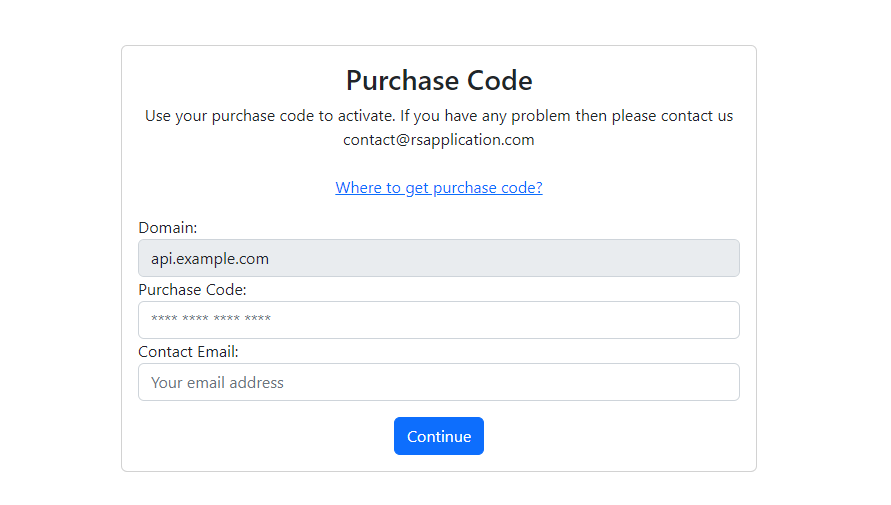This image is a screenshot taken against a white background, which features a centered interface for entering a purchase code. The screen is outlined in gray and displays a structured layout. At the top, bold black text reads "Purchase Code." Below this heading, a subtext instructs the user: "Use your purchase code to activate. If you have any problem, then please contact us. Contact at rsaapplication.com."

Underneath this instructional text, there is a blue, underlined link labeled "where to get purchase code." Following this, there is a section for domain input, featuring a gray-outlined box containing the text "api.example.com."

Below this domain section, the interface asks for the "Purchase Code," and provides a secure input box filled with asterisks for privacy. Subsequently, another labeled field requests a "Contact Email," with a gray-text placeholder reading "your email address."

Towards the bottom center of the interface, a prominent blue button with white text invites the user to "Continue." The entire page is bordered by a thin gray line on all sides, giving it a neatly framed appearance within the screenshot.